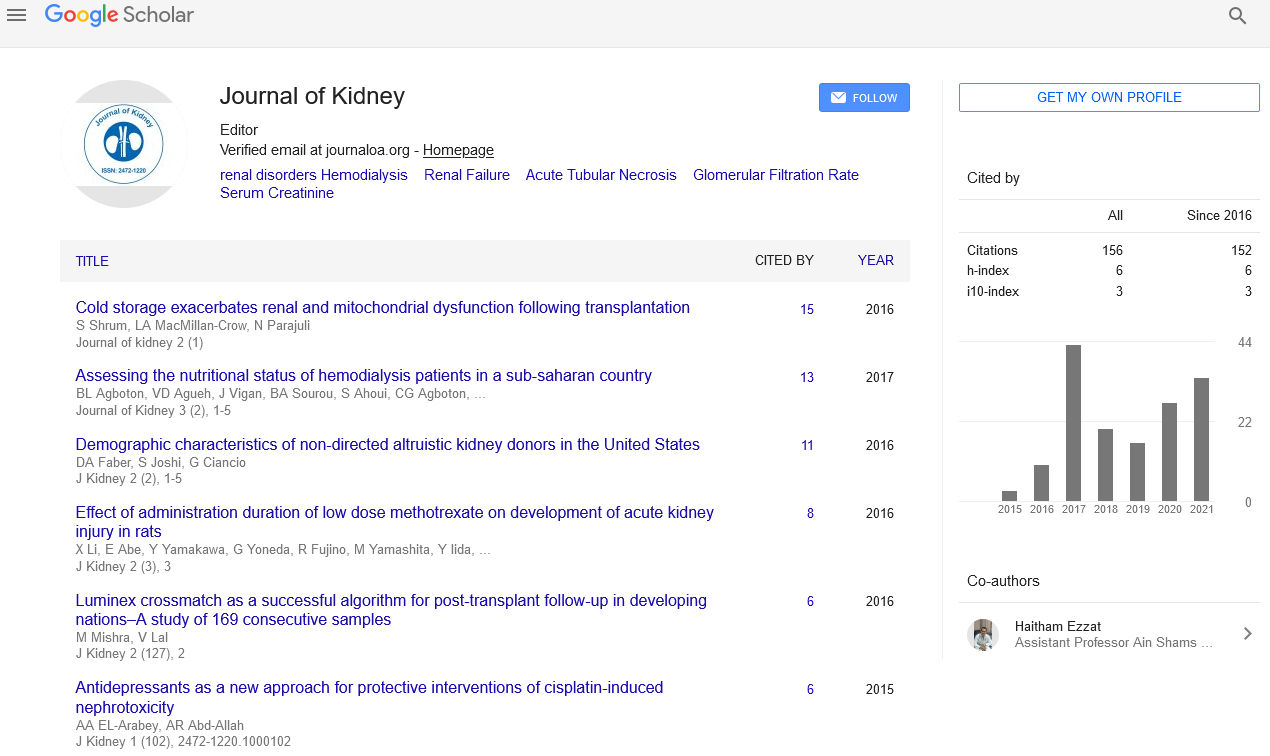This is a screenshot from Google Scholar showcasing a profile related to "Journal of Kidney." The recognizable Google logo displays its signature colors: blue, orange, red, and green. Below the logo, "Scholar" appears on a gray bar stretching across the page. The profile includes "Journal of Kidney" written in black text, accompanied by a circular image featuring teal writing and gray sections at the top and bottom, labeled as "Editor."

The profile further mentions a verified email at journalmake.org. Keywords associated with the profile include "renal disease," "disorders," "hemodialysis," and "renal failure," referenced under the header "All about kidneys," written in purple text at the top. Below the title, various resources and publications related to the Journal of Kidney are listed. 

In the upper-right corner, a blue bar featuring an envelope icon is visible. To the right, there is an option for "Get my own profile." Metrics such as "Cited by," "All," and "Since 2015" are present, along with citation indexes like "h-index" and "i10-index." A bar graph illustrating citation counts from 2015 to 2021 shows varying heights, peaking at 44, with the smallest being around 2. There is also a mention of co-authors, including a reference to "Assistant Professor Annie Shams."